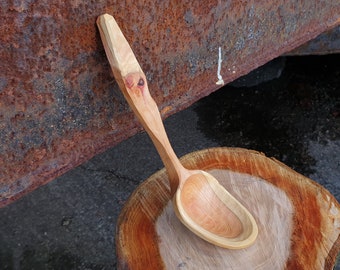This is a detailed and reflective photograph of a crudely carved wooden spoon with an uneven handle and a deep, curved scoop. The spoon, made from a light brown piece of wood with a darker brown center and a visible tree ring, sits precariously against a rusted steel beam. The handle of the spoon also features a noticeable knot. Beneath the spoon is a circular cutout of what appears to be a tree trunk, characterized by its thick brown ring encircling lighter tan wood. The scene is complemented by a marble or stone texture with orange and light gray hues, creating a visually cohesive aesthetic. The entire composition is overlaid with a thin, watery surface, adding a reflective quality to the image and blending the colors of the wooden spoon, rusted beam, and decorative underlay.